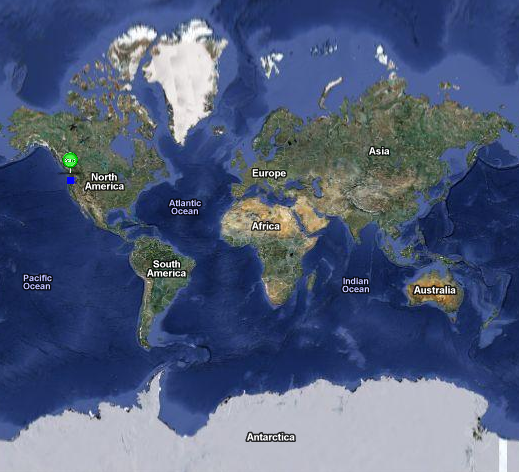This image displays a meticulously drawn map of Earth, presented on a flat surface. The map, known as UKE, comprehensively illustrates the entire world as we understand it, complete with detailed labels. It includes all the continents: North America, South America, Africa, Europe, Asia, and Australia. The map also delineates the major oceans, specifically the Pacific Ocean, the Atlantic Ocean, and the Indian Ocean. Toward the bottom, the Arctic region is depicted in a solid white color. This map is typical of standard world maps one might encounter in educational settings or general reference. On the left side, within the North American region, there is a small blue square marked with a pin, likely indicating a specific location, possibly where an individual or point of interest is situated.